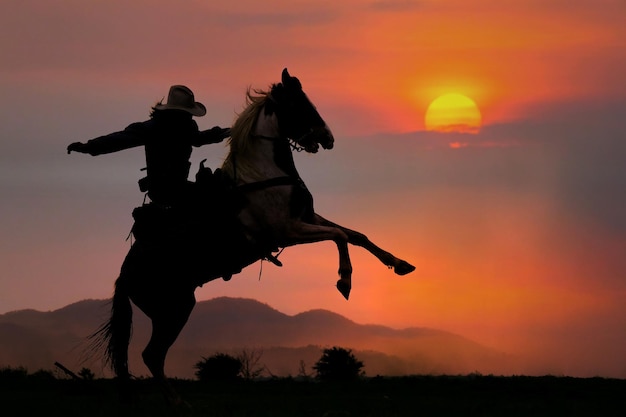In this striking photograph, a cowboy is dramatically silhouetted atop a rearing horse, its front legs high in the air while it balances on its hind legs. The cowboy, wearing a wide-brimmed hat, grips the horse's reins with his left hand as his right arm extends behind him, intensifying the sense of motion. Although the details of both the rider and the horse are obscured in silhouette, the horse's mane and the person's hair flow backward, capturing the dynamic energy of the scene. 

The backdrop is a breathtaking sunset, painting the sky in a gradient of orange, pink, purple, and blue hues. The deep yellow sun peeks from behind a low-hanging, partially obscuring cloud, adding a golden glow to the scene. Silhouetted mountain ranges stretch across the horizon, framing the dramatic moment. In the foreground, the flat terrain is punctuated by the dark silhouettes of two bushes, emphasizing the wide-open landscape. This image, with its vivid colors and powerful contrasts, captures the raw beauty and spirit of the cowboy's world.